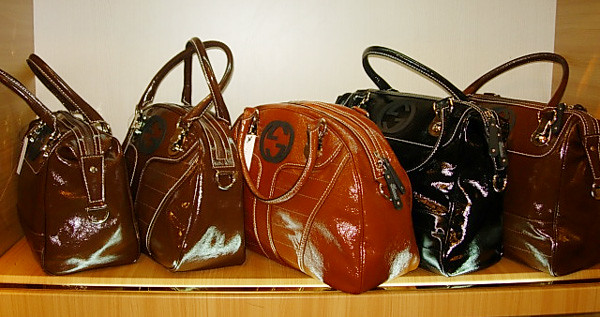The image depicts a wooden bookshelf-like display mounted against a pristine white wall, showcasing an elegant collection of five luxurious handbags. Each handbag exudes a glossy, high-end finish and comes in a spectrum of rich colors including shiny brown, dark brown, maroon, and black.

Starting from the left, the first handbag is a glossy brown bag with silver trim, adorned with a distinctive white tag on its front. It features unique looped handles. Next to it is a dark brown handbag which has white outlines resembling pockets, with its handles intricately interwoven. The third bag is maroon, boasting a black emblem with a central design, accentuated by black tassels and a silver tag hanging from its side. The fourth handbag is a black bag with brown handles and a prominent brown emblem at the front, featuring some text. Lastly, the fifth bag is a dark brown color, highlighted with gold buckles on its front. Each handbag on the shelf not only showcases exquisite craftsmanship but also hints at opulence and luxury.